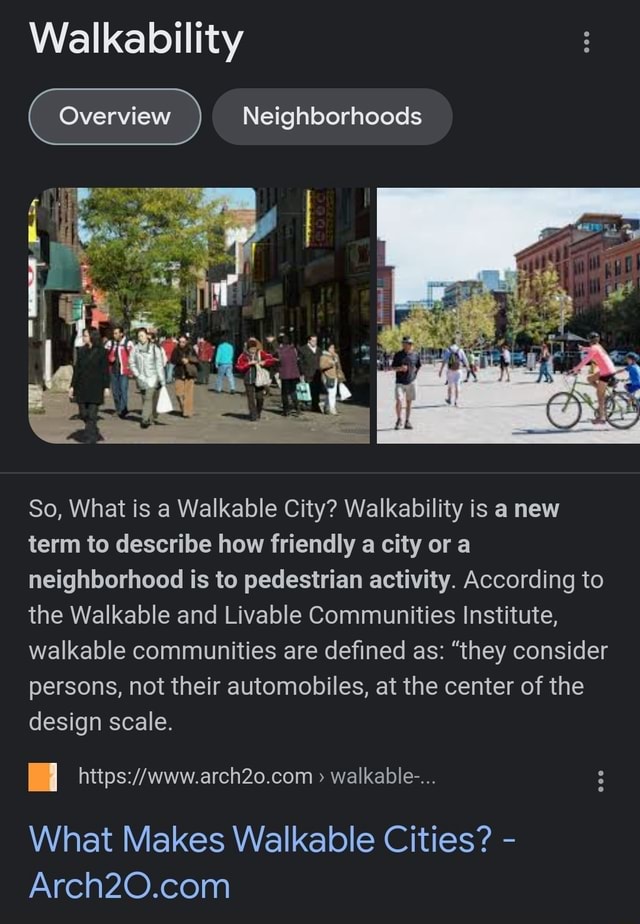The image is a screenshot from a Google search performed on a mobile device. The search results pertain to the topic of "walkability," which is prominently displayed as the title of the search page. Beneath this title, there are two interactive buttons: one labeled "Overview" and the other "Neighborhoods." The page includes several thumbnail images that exhibit scenes of walkable urban areas, highlighting pedestrians and cyclists in environments seemingly designed for foot traffic.

Directly beneath the thumbnail images is a textual excerpt from an article hosted on arch20.com, which elaborates on the concept of walkability. The text states, "Walkability is a new term to describe how friendly a city or a neighborhood is to a pedestrian or to pedestrian activity. According to the Walkable and Livable Communities Institute, walkable communities are defined as those that consider persons, not their automobiles, at the center of the design scale." The images accompanying the text support this description, depicting urban scenes with numerous pedestrians and minimal car presence, emphasizing the pedestrian-friendly infrastructure of these communities.